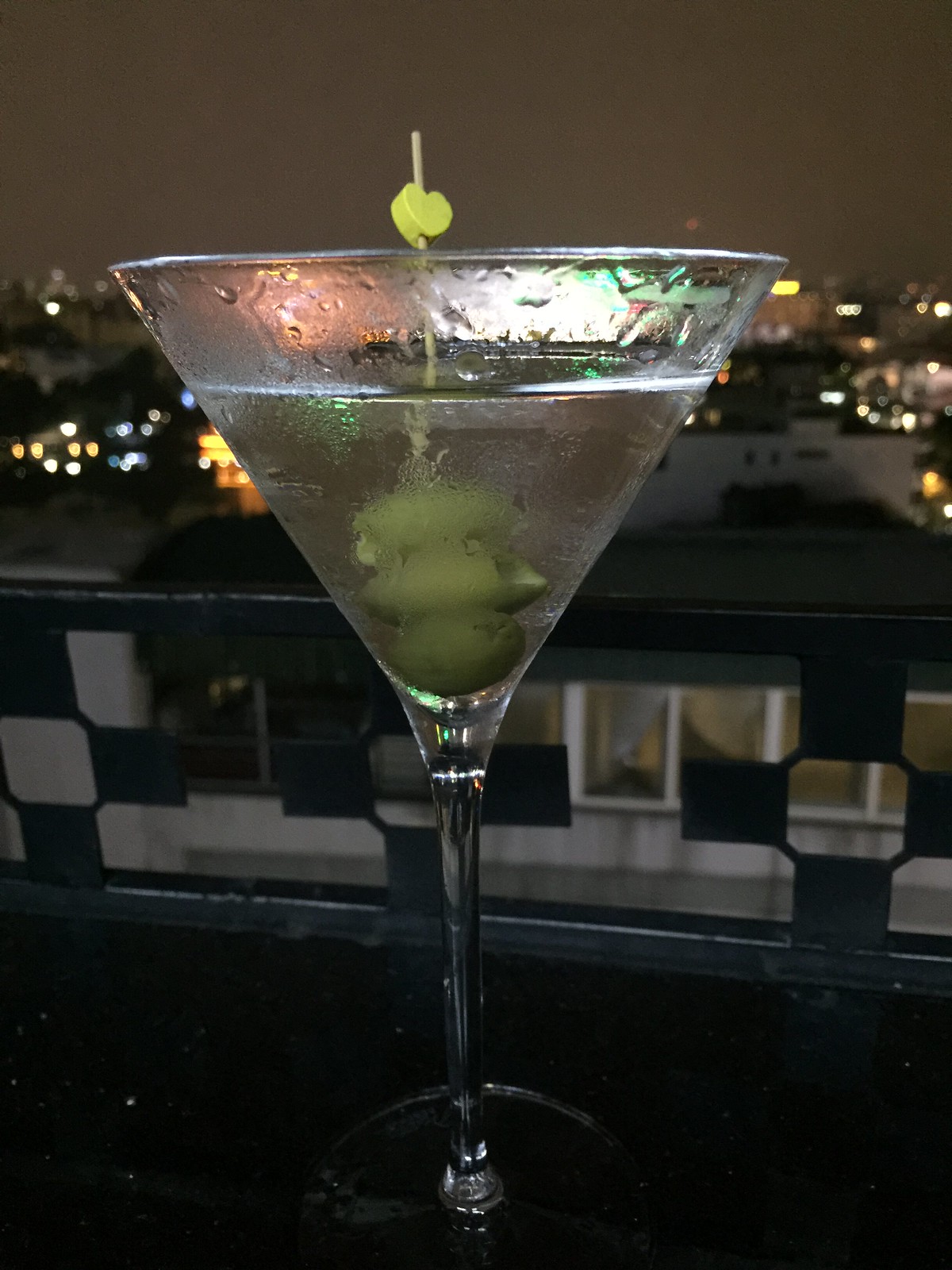This is a tall rectangular image showcasing a martini glass filled with a clear liquid, positioned on a dark surface. The martini glass extends nearly to the top of the image, featuring condensation that hints at its chilled nature. Inside the glass, three dull green olives are stacked on a toothpick, which protrudes from the glass and is adorned with a light green, heart-shaped bead. The backdrop is a dark gray nighttime sky, with a illuminated city skyline unfolding beneath it. The lower half of the image reveals what seems to be a glass barrier, likely part of a balcony, featuring a square-shaped design pattern. Beyond this barrier are the lit windows of a white building with a black rooftop, contributing to the intricate tableau of city lights in the background.